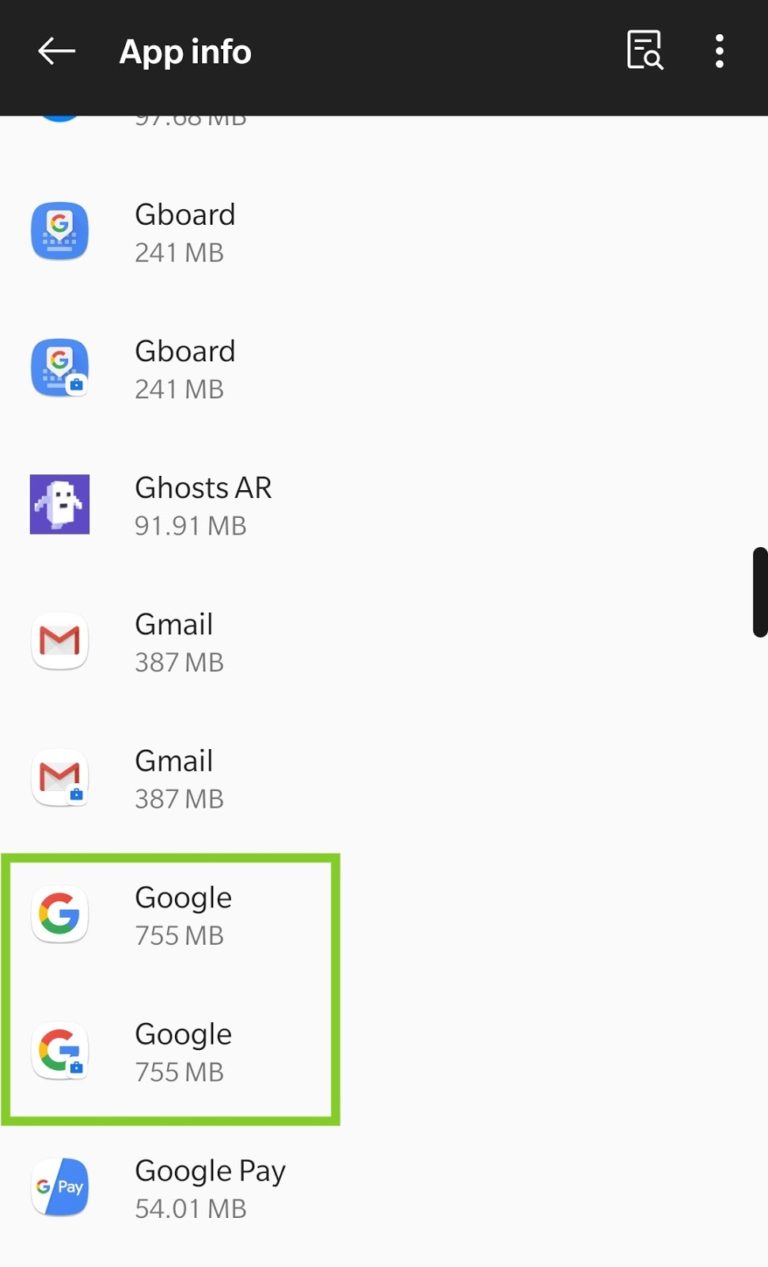This image depicts a screenshot of a smartphone displaying the 'App Info' settings. The screen is overlaid with a prominent diagonal watermark saying "Watermark," running from the top left to the bottom right. The vertical list of apps includes multiple entries of Gboard, GhostAR, Gmail, and Google. Two Google app entries are boxed within a green outline. Additionally, there is another overlay watermark at the bottom of the image that states "This image is protected." Underneath the green outline, the list continues with Google Pay. The image suggests that a person is reviewing their list of installed apps, which includes duplicate entries, although it is not clear why this inspection is taking place. The watermarks indicate that the image is protected, possibly added by the creator or Google to prevent unauthorized use.